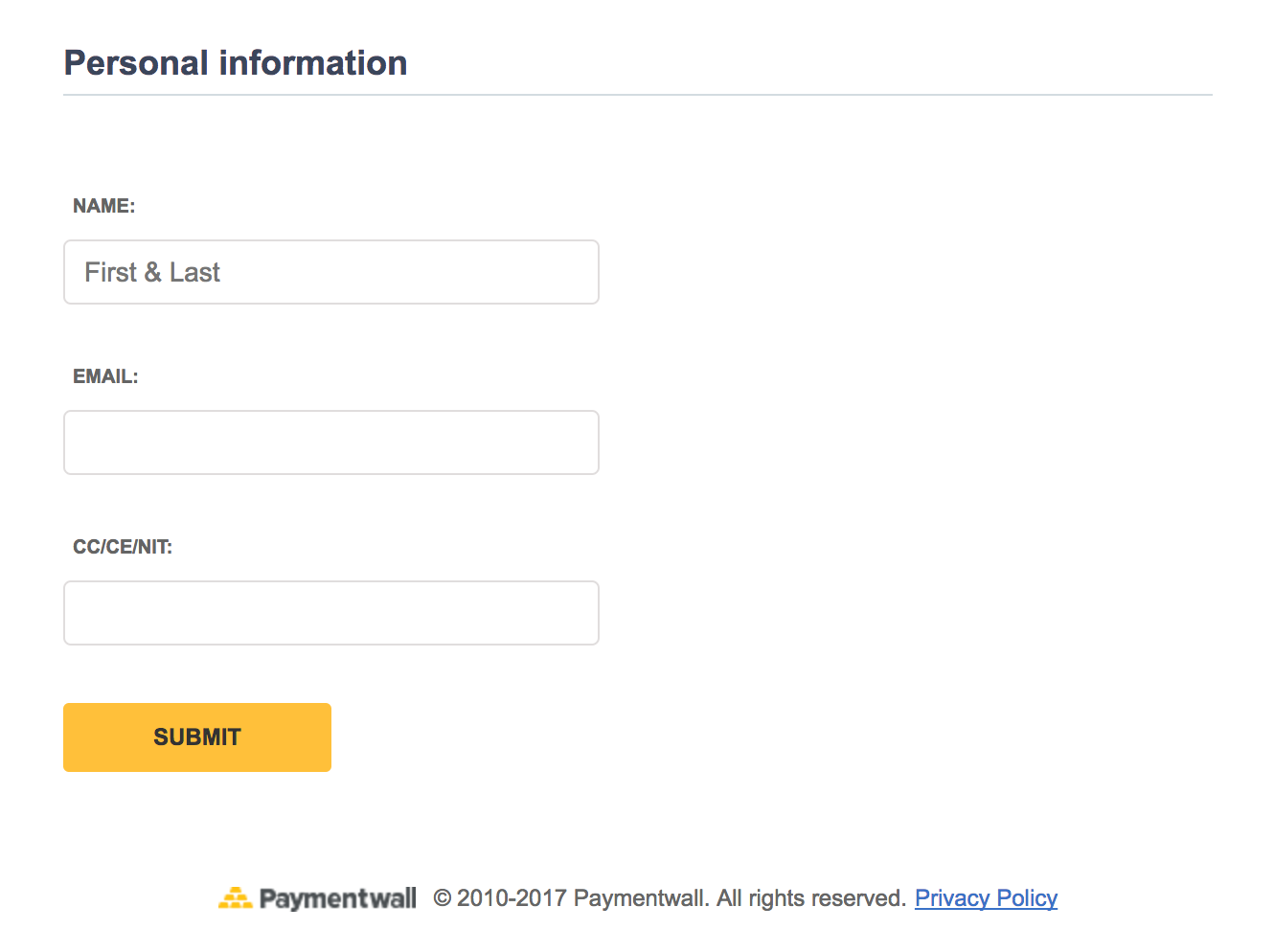This image features a form set against a white background. At the top of the form, the words "Personal Information" are prominently displayed, followed by a long gray line underneath. Below this, there are fields to input personal details:

1. "Name" field, with a white box outlined in gray to enter both first and last names.
2. "Email" field, again with a gray-outlined white box for entering an email address.
3. "CC/CE/NIT" field, with another gray-outlined white box for additional information.

Towards the bottom, there is a distinctive yellow "Submit" button for submitting the information. Beneath the button is a small, visually appealing graphic: six small yellow dots arranged in a pyramid shape. This is accompanied by the text "Paymentwall" next to it. Additionally, a copyright notice reads "© 2010 to 2017 Paymentwall. All rights reserved". Finally, at the bottom-right corner, there is an underlined, blue "Privacy Policy" link, indicating further information about their privacy practices.

This form is clearly designed to collect personal information and features a bright yellow submit button for ease of submission.